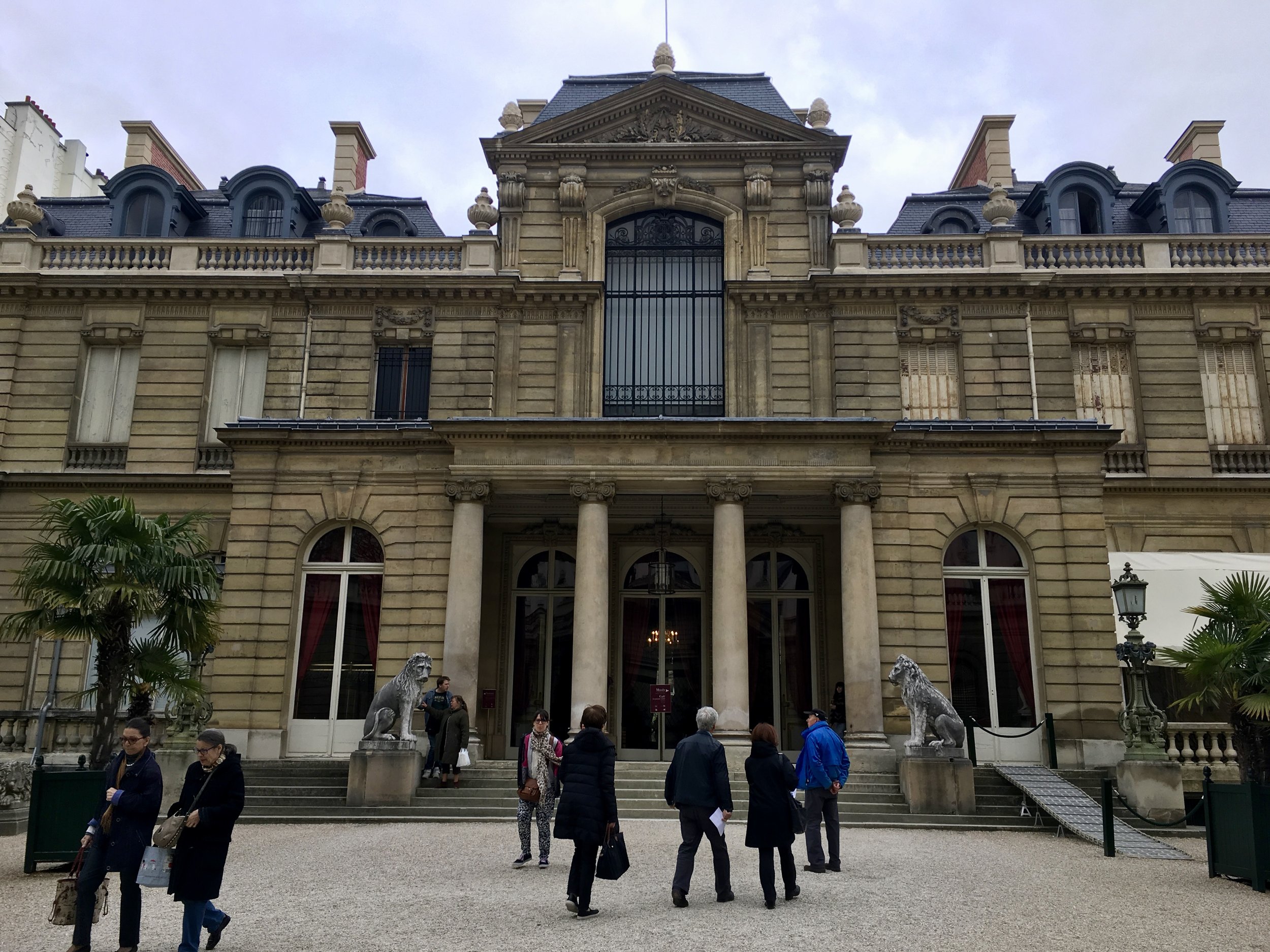This photograph captures a grand, classical-style building made primarily of light brown stone and brick. The three-story structure exudes an air of officialdom, reminiscent of late 18th to early 19th-century architecture, possibly a government or institutional building. The facade is adorned with four tall, elegant columns flanking a wide series of steps leading up to a prominent entrance.

Lion statues stand guard at the base of the staircase, adding to the building's grandeur. The front entrance is characterized by three tall vertical windows, two of which flank the large central window that doubles as a door. Above the columns and stairway, the building features additional decorative elements, including elaborate structures and railings on the roof, which reveal small statues and intricate designs.

The second floor boasts vertical rectangular windows with gray casements, nearly reaching from ceiling to floor. Centrally located above the main entrance is a large arched opening, suggestive of a balcony, although no balcony is visible. This is topped by a high raised gabled peak. Flanking this central structure, the third story features a mansard roofline punctuated by dormered windows with arched tops and wide fireplace chimneys between them.

In front of the building, a wide paved cement walkway is bustling with people. Some are walking towards the entrance, while others are walking away or standing on the steps. The individuals are dressed in modern, professional attire, suggesting that this is a place of business or an official institution. The scene is set during the winter or in cold weather, as indicated by the clothing worn by the people. 

Overall, the combination of architectural grandeur and the busy, modern crowd creates a vivid juxtaposition, emphasizing the building's historical significance and ongoing relevance.